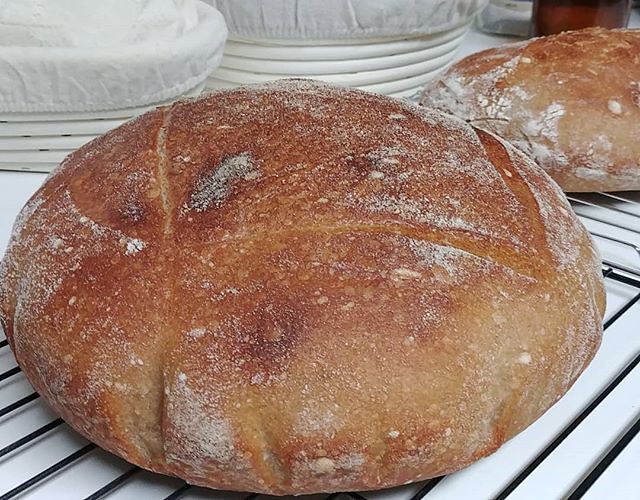This photograph captures two freshly baked pastries, prominently set on cooling racks atop a pristine white table. The pastries, one round and the other slightly oval, are generously dusted with flour or powdered sugar, giving them an inviting, homemade appearance. The bigger pastry, resembling a giant bun, is adorned with delicate creases across its top, hinting at its fluffy, airy texture, likely achieved with yeast. In the backdrop, there are various white plates or bowls, some covered to keep them clean, indicating a meticulous baking environment. Additionally, a brownish glass or water bottle is partially visible, adding a subtle touch to the scene. The overall lighting is excellent, possibly suggesting the photo was taken in a well-lit kitchen or an outdoor venue.